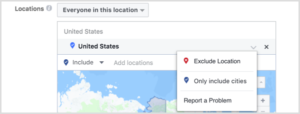This image appears to be a blurry screenshot set against a large white background. In the upper left corner, the word "Locations" is displayed in black text, accompanied by a small eye icon enclosed in a gray circle to its right. Beside this, there is a pull-down box labeled "Everyone in this location."

Below this section, a portion of a map is visible. Though it lacks clearly discernible details, the map features a blue area primarily at the top, transitioning to white and green regions. Additionally, there's a blue outline around a small gray area in the center of the map.

Overlaid on this map is a small box containing the text "Exclude location," "Only include cities," and "Report a problem." To the left of "Exclude location" is a red teardrop shape, while a blue teardrop shape is situated to the left of "Only include cities."